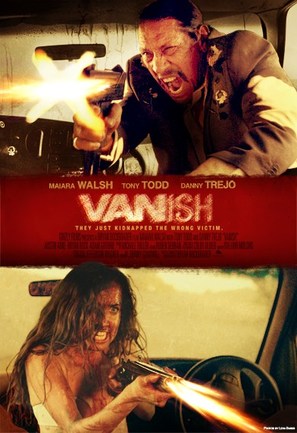This is an action-packed movie poster for the film *Vanish*. Dominating the center is a red block with the movie's title, *Vanish*, prominently displayed in large white letters. The tagline below ominously reads, "They just kidnapped the wrong victim." Above the title, the names of the main actors—Maria Walsh, Tony Todd, and Danny Trejo—are listed.

In the top third of the poster, Danny Trejo commands attention with an intense, action-filled scene. He is depicted inside a car, aiming and firing a submachine gun with a fierce expression, mouth agape as if yelling. His hair is pulled back, and he is wearing a brown coat, with a bright light illuminating his right hand.

At the bottom of the poster, a woman with long brown curly hair, likely portrayed by Maria Walsh, appears equally intense. She is also inside a car, fiercely shooting a gun that emits a burst of fire. Her face is dirtied, and she wears a white tank top, gritting her teeth in determination.

Overall, the vivid imagery and bold text emphasize the high-stakes action and drama at the heart of *Vanish*.